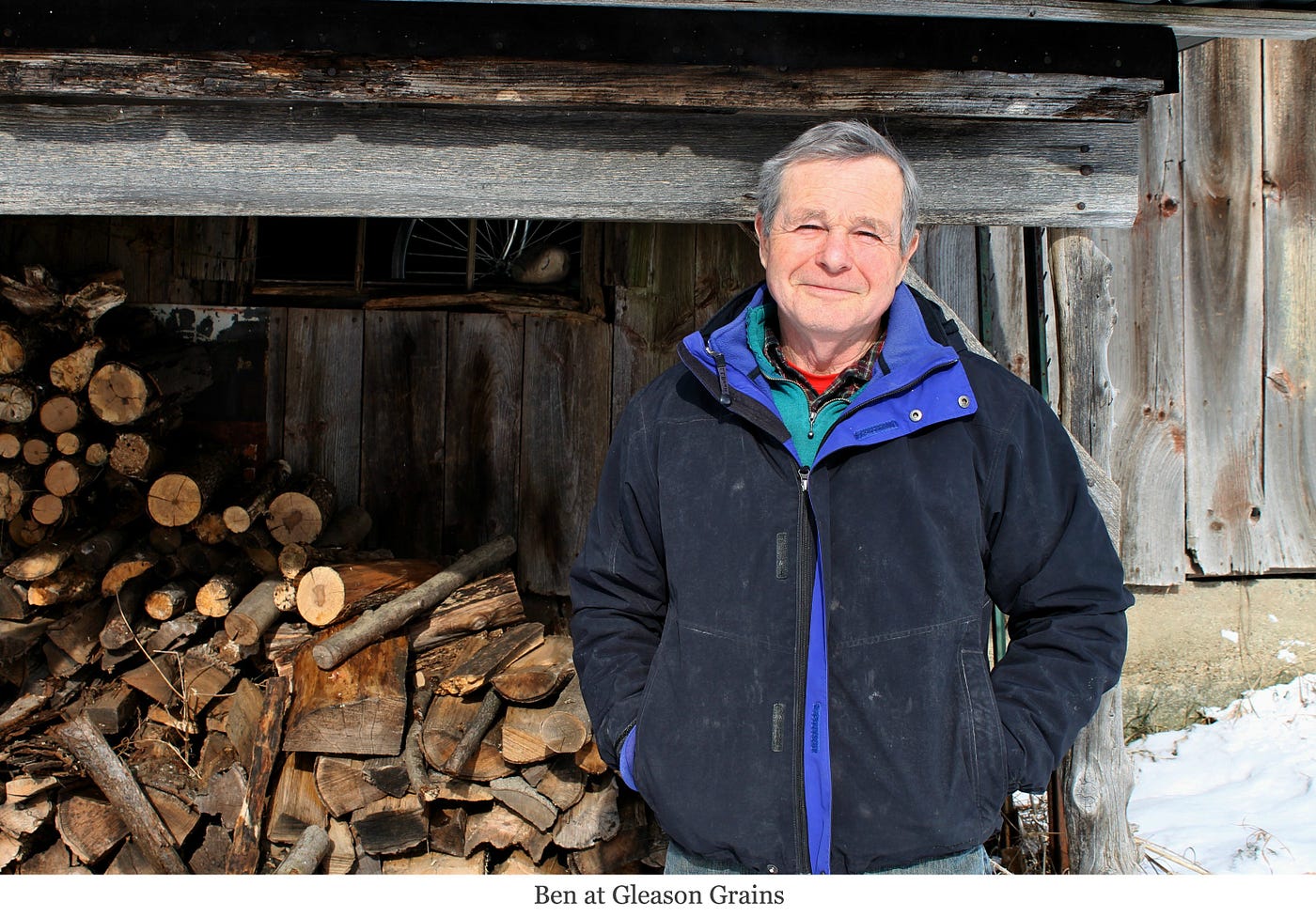In this pleasant outdoor winter scene, an older man named Ben, around 75 years old, stands smiling in front of a pile of chopped wood under a wooden shed roof. He wears a black jacket with blue lining, which has snaps and is mostly zipped up, revealing a teal undershirt and a red t-shirt underneath. His gray hair and beaming smile stand out against the backdrop of a rustic old barn and snow-covered ground. The woodpile behind him is somewhat disarrayed, with logs that have tumbled down. The caption at the bottom reads, "Ben at Gleason Grains."